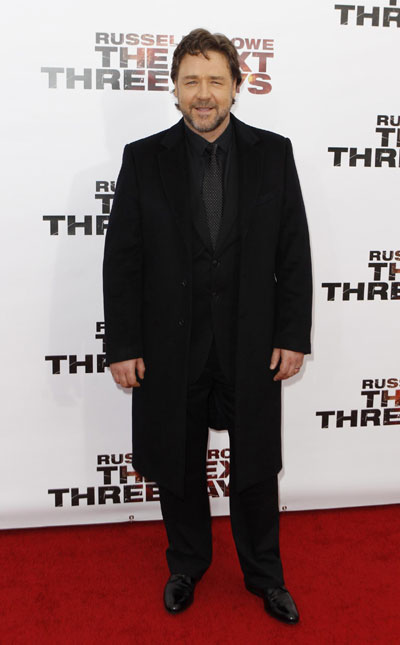This is a color photograph of the famous actor Russell Crowe, captured as he walks the red carpet for the premiere of his movie, seemingly "The Next Three Days." The full-body shot shows Crowe dressed in an all-black ensemble, featuring a knee-length dark coat, a matching shirt and tie, black pants, and shiny black shoes. His hands, which are visible from the sleeves, rest naturally at his sides, with a ring noticeable on his left ring finger. Crowe's short, wavy hair is neatly combed, and he wears a closely shaved goatee that integrates with his mustache. He appears to be slightly squinting, likely due to the camera lights, and he has a subdued smile on his face. The backdrop behind him reads "Russell Crowe" and "The Next Three Days," though part of the text is obscured by his figure. His stance and expression suggest he has paused to pose for the media, a common scene at red carpet events.